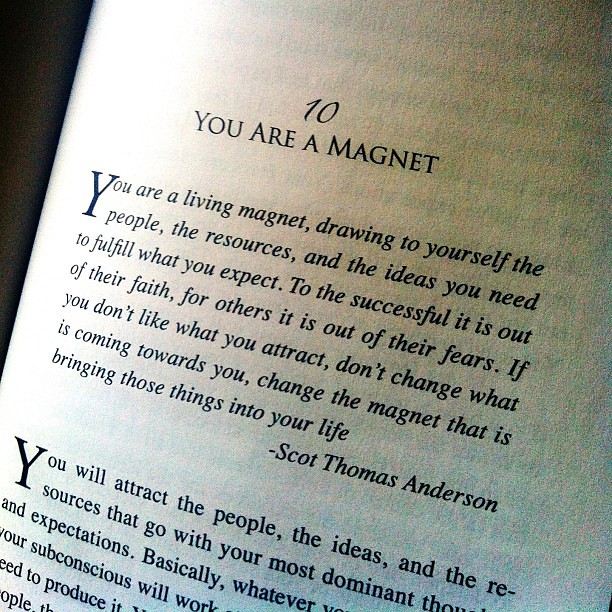This image depicts a page from a book written in black italic font on a white background. At the top of the page, in larger font, it reads, "10. You are a magnet." The text continues with an inspirational message by Scott Thomas Anderson: "You are a living magnet drawing to yourself the people, the resources, the ideas you need to fulfill what you expect. To the successful, it is out of their faith; for others, it is out of their fears. If you don't like what you attract, don't change what is coming towards you. Change the magnet that is bringing those things into your life." The page then transitions into another paragraph, but the image cuts off, leaving the text incomplete. It begins: "You will attract the people, the ideas, and the resources that go with your dominant..." and trails off. The photo captures the entire page, angled slightly, suggesting it comes from a motivational text.